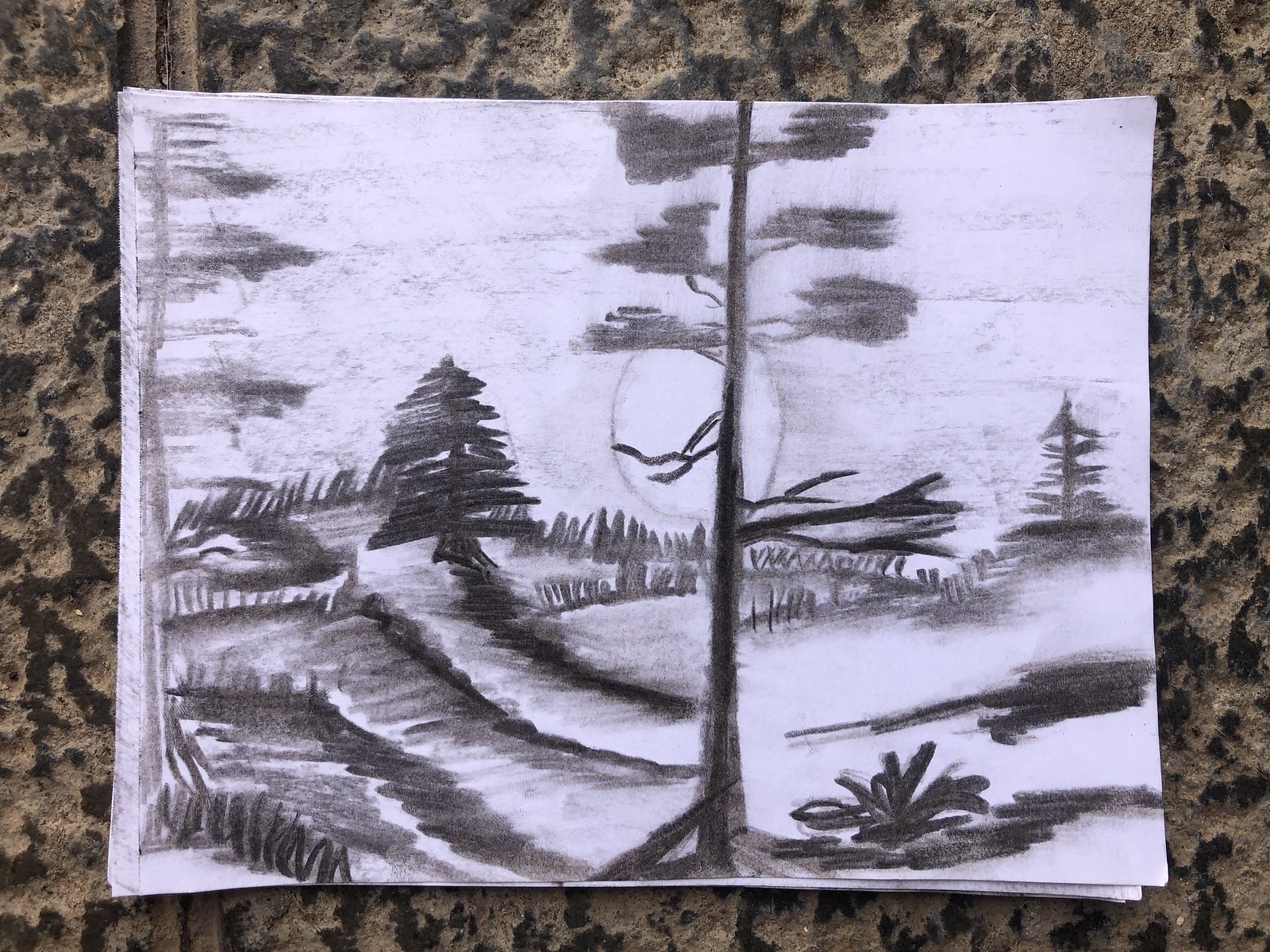The image displays a black and white charcoal drawing on a standard-sized sheet of paper, resting atop a quartz countertop with an intricate brown-gray design. In the drawing, a prominent tall tree stands in the center, with a mix of branches—some baren near the bottom and a few with sparse leaves towards the top. Surrounding the central tree, there are additional trees, including a couple that resemble Christmas trees, all depicted with broad, expressive charcoal strokes. The landscape features rolling hills and scattered vegetation, with the ground depicted through a combination of stark white spaces and dense black scribbles representing grass. In the distance, the sun peeks fully over the horizon, adding depth to the textured scenery.